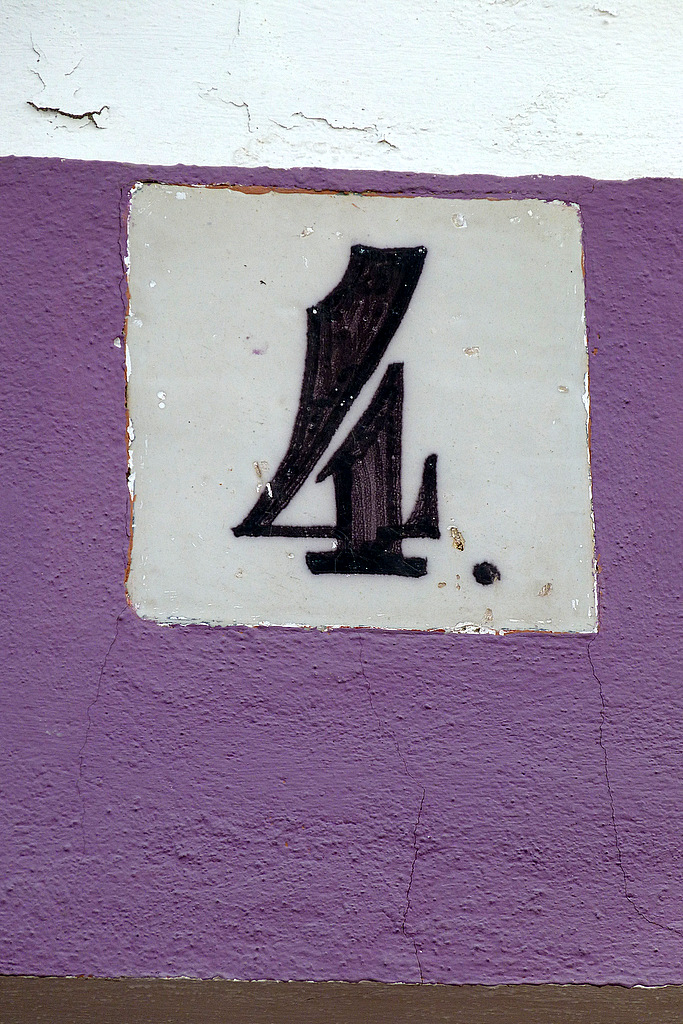In this close-up portrait-mode photograph, the focus is on a large, stylized black number 4 followed by a period, painted with wide strokes that give it a calligraphic flair. The number 4 is situated on a gray concrete or linoleum tile, which appears inset into a rougher, predominantly deep eggplant purple wall. The tile's smooth, creamy-gray surface contrasts sharply with the textured, cracked purple wall. The wall itself features a white stripe at the top, which is peeling to reveal the purple paint beneath, and a narrow brown strip at the bottom, which may be part of a wooden door frame. The lighting suggests this scene is outdoors, likely captured during daylight hours.